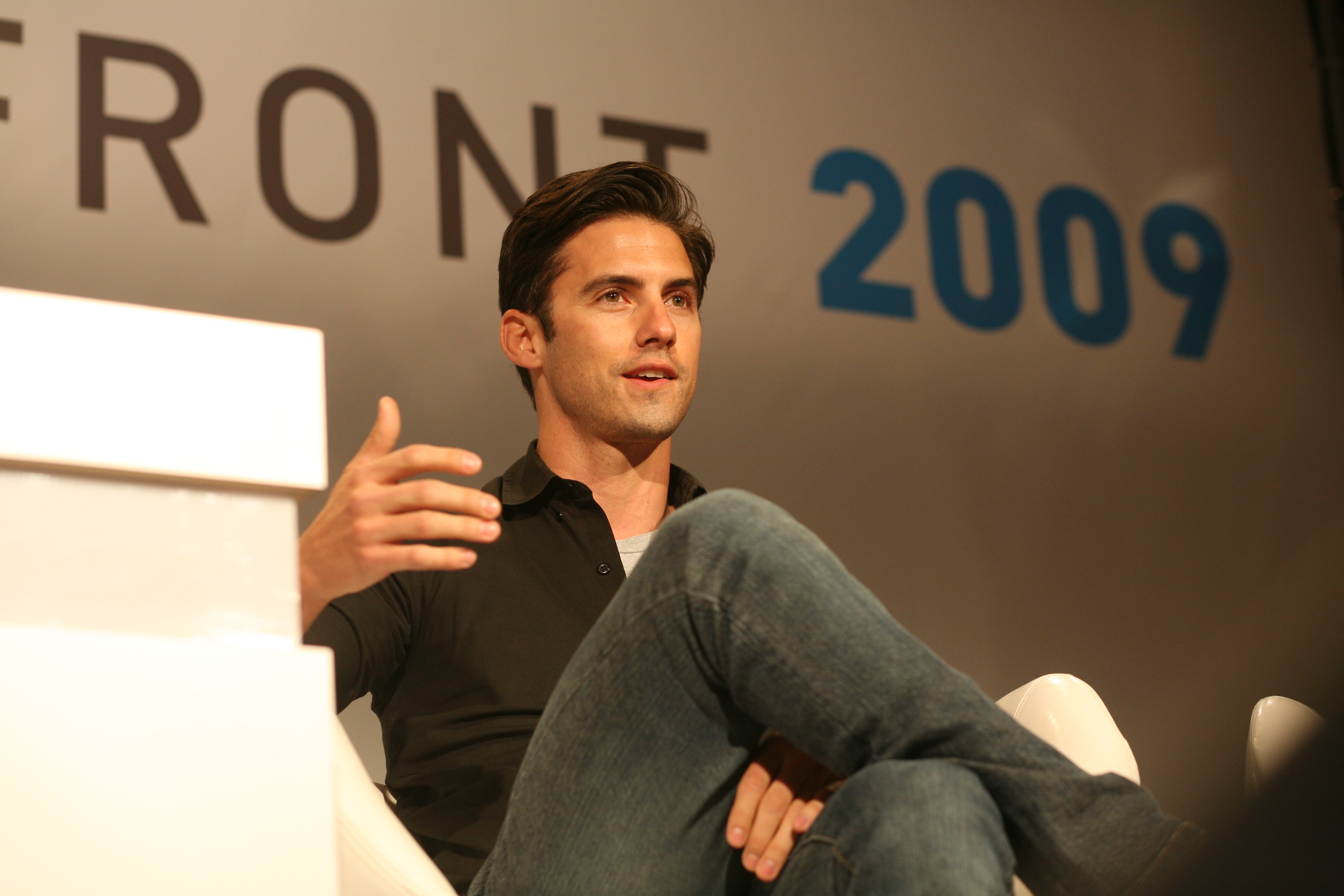In the photograph, a person is seated on a low, plastic-looking armchair positioned centrally on a stage. The background is a solid white wall with text that reads "Front 2009," where "Front" is in black font and "2009" is in blue font. To the left of the person, there is a partially visible white podium. The individual, who appears to be speaking at a conference or convention, is dressed in dark blue jeans and a black long-sleeve button-up shirt with the sleeves rolled up. Underneath, they have a gray short-sleeve shirt. Their black hair is styled and gelled to sweep to the right. The person's right leg is crossed over their left knee, their right hand is raised in a speaking gesture, and their mouth is partially open as if addressing an audience.